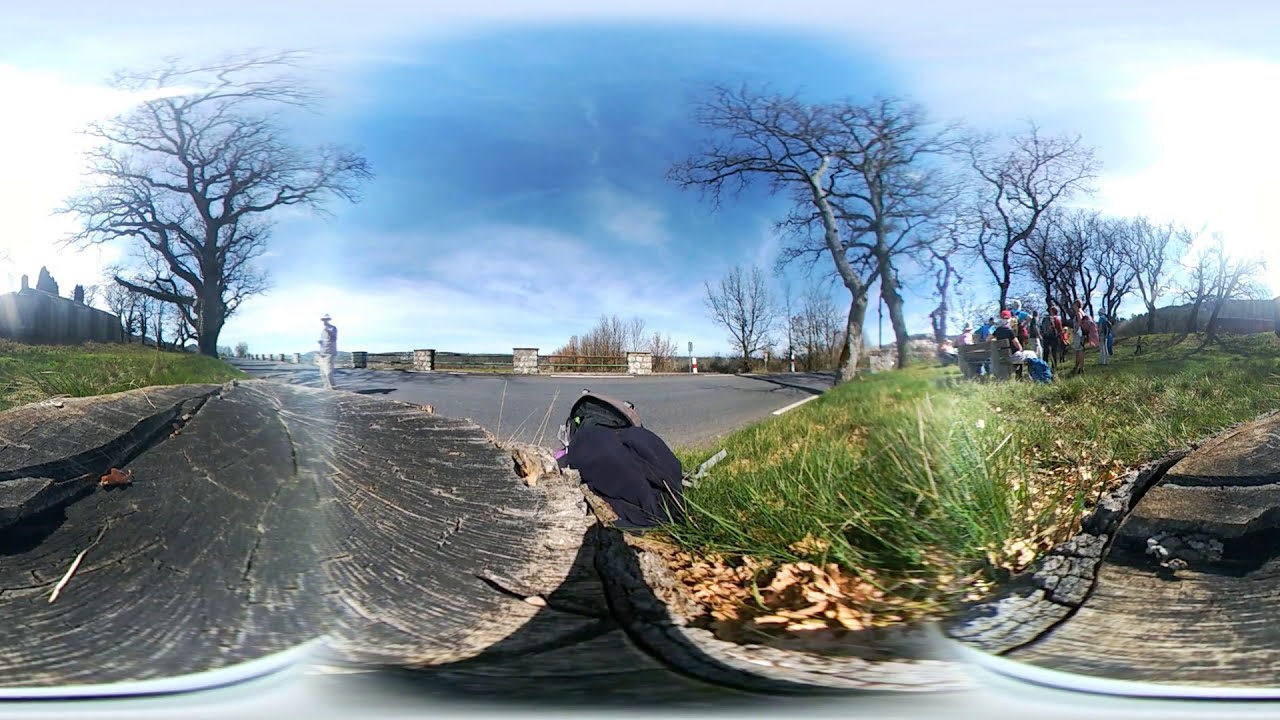The photograph depicts a panoramic outdoor scene, primarily dominated by nature, despite some distortion. The foreground features a massive, halved tree trunk with visible black bark, seemingly serving as a makeshift stand for the camera. The landscape appears in late autumn or early winter; the trees are barren, devoid of leaves. A blue sky with a smattering of clouds provides a backdrop, casting natural light across the scene.

At the center and slightly to the right, a group of well-dressed people, bundled in winter coats, suggest a cold day. One central figure is particularly noticeable, wearing a full winter coat with a fur hood. These individuals seem to be gathered casually, possibly for a picnic, in a park-like setting, with some of them seated around a bench surrounded by greenery. Grass is present, albeit patchy and dying in places, and some oval areas show brown foliage indicative of the season.

To the left, another figure stands on a concrete area resembling a parking lot, contrasting with the natural setting to his right. Beyond the group of people, in the distance, faint outlines of buildings are interspersed among the trees. The scene, rich in colors such as blue, white, gray, brown, green, orange, and tan, captures a cold yet sunny day in what appears to be a public park.